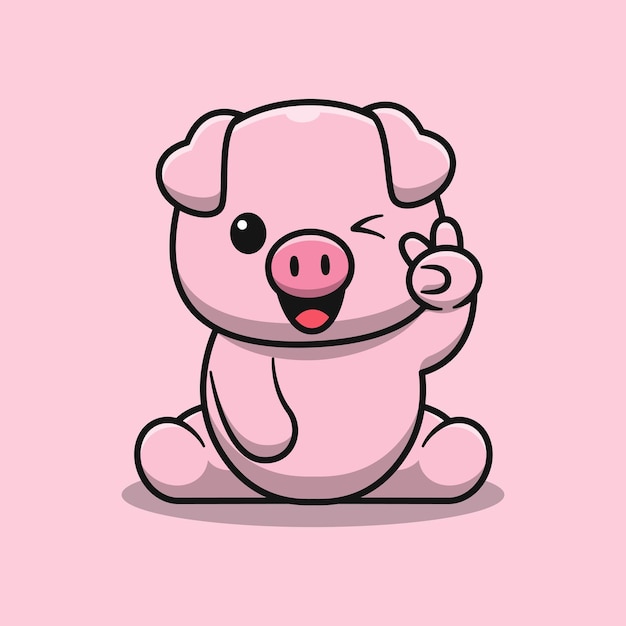In this charming cartoon illustration, a cute little pink piglet is the central focus, set against a matching pink background. Outlined in black, the piglet is depicted with one shiny black right eye featuring a small white pupil and a left eye winking as a squinty black line. The pig's pink snout is large and prominent, while its open mouth reveals a tiny red tongue against a black interior. The piglet's left hoof is raised, forming a peace sign with two fingers, while its right paw rests downward. Sitting comfortably on the ground with its legs splayed out to the sides, the piglet's floppy ears hang endearingly towards its face. The whimsical details of the black outlines and the piglet’s charming expression contribute to the overall adorable and playful essence of the image.